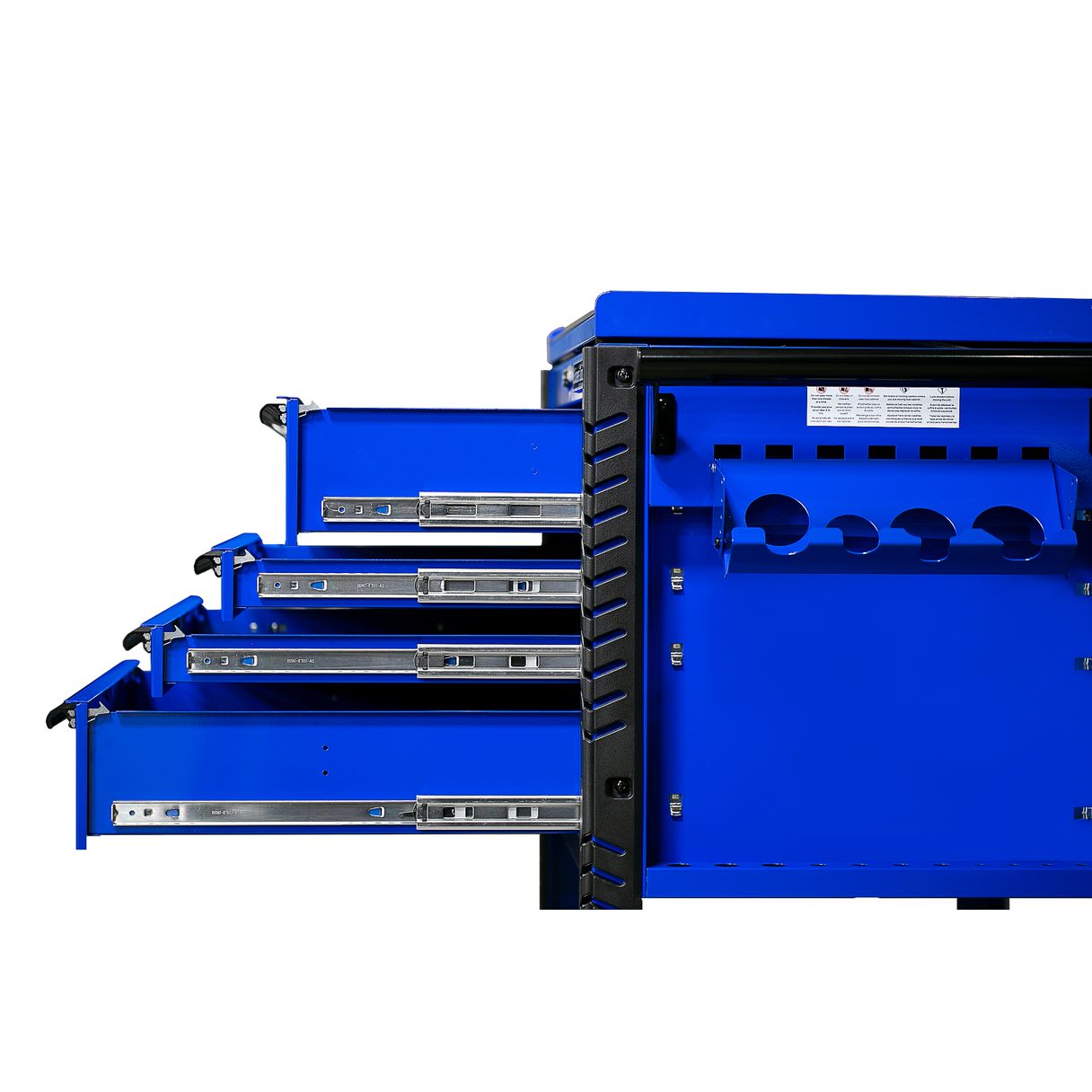This image showcases a computer-generated drawing of a blue industrial equipment piece set against a stark white background. The focal point is a large cube-shaped structure, resembling a mechanics toolbox or possibly an office printer. The box is highlighted with a bold black border and stands on sturdy black legs. The side view reveals four blue drawers, with each progressively pulled out further from top to bottom. The top and bottom drawers are notably larger, sandwiching two thinner middle drawers. These drawers feature shiny silver or chrome sliders and dark-colored pulls, providing a contrast against the bright blue of the drawers. Additionally, a small white plaque on the main body bears black lettering, though the text is unreadable due to its small size. Rectangular holes are visible near the top on the side, adding to the design detail.